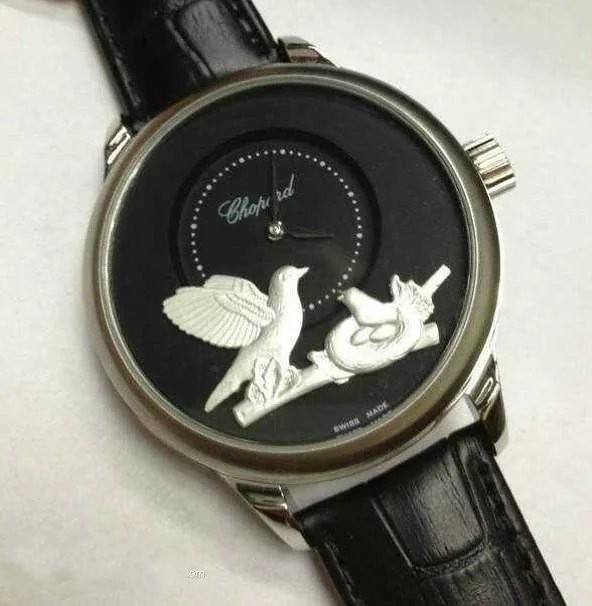A close-up image of a sophisticated watch with a striking design. The watch face is adorned with two intricate cameo-style images in white, depicting a bird and her nest, set against a black background. The watch features a small inner dial with a pair of hands. Encircling the face is a silver bezel that adds a touch of elegance. The watch is complemented by a premium leather strap with silver fittings and is equipped with a large white winding knob on the right-hand side.